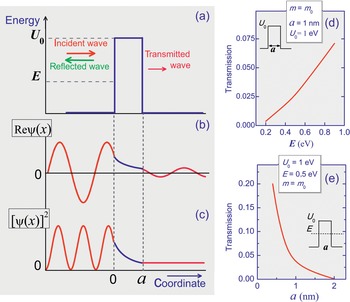The image comprises five detailed scientific graphs with gray backgrounds on a white canvas, labeled A through E, each illustrating different aspects of energy and transmission waves. 

On the left, three prominent graphs (labeled A, B, and C) are presumably oscilloscope traces depicting wave behavior over time or distance. Graph A, the largest, demonstrates a square wave signal, with the y-axis labeled 'Energy.' The x-axis, although unlabeled, is inferred to represent time or distance. Distinctly, the graph highlights 'incident wave' in red, directing right; 'reflected wave' in green, pointing left; and a 'transmitted wave,' also moving right but denoted by a blue square wave. 

Graph B appears intricate, beginning with an incident sine wave in red that notably decays at the interference point—corresponding to the blue region from the square wave in Graph A—resulting in a diminished sine wave pattern post-interference. The y-axis here is tagged 'Re ψ/n x closed/n,' representing a scientific variable. Graph C continues the sine wave analysis, solely in the positive domain with a higher frequency, exhibiting similar decay patterns but transitioning to an unmodulated transmitted wave. This graph’s y-axis is identified as 'ψ/n x closed/n squared.'

On the right, two smaller graphs (labeled D and E) focus on transmission metrics. Graph D features a red line ascending, while graph E exhibits a red line descending and curving. Both graphs contain intricate scientific symbols and are indicative of energy flow variations, highlighting the energy's ascending and descending transmissions respectively.

Overall, the graphs employ red and blue lines to distinguish different wave measurements and are designed with legends to decode the scientific variables, underscoring the meticulous nature of energy and wave transmission analysis detailed in this image.